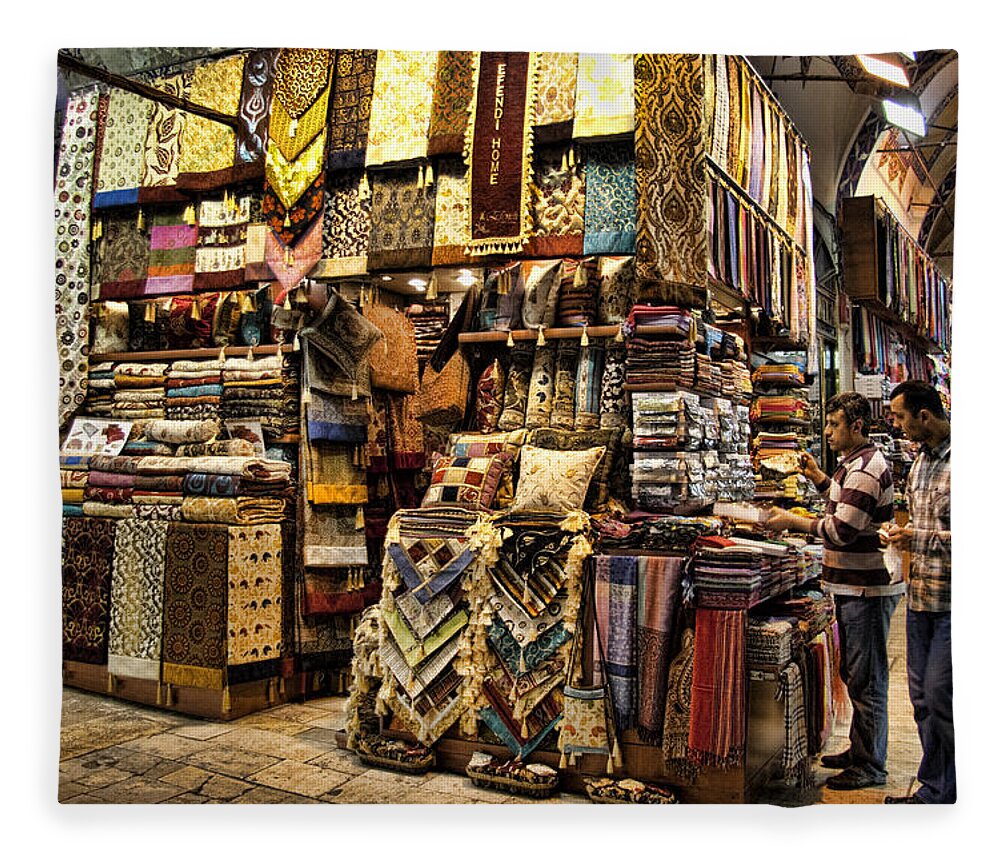The image is a vibrant, color photograph of an outdoor carpet market, likely located in India. Dominating the scene are walls of carpets, tapestries, and other textiles that stretch from the top of the frame to the bottom, creating a seemingly endless array of colorful patterns and textures. To the bottom right-hand corner of the image stand two men of Indian descent, both dressed in jeans and striped shirts. One man is engaged, touching the textiles, while the other looks at the samples. The market layout includes not just piled carpets but also hanging tapestries, pillows, and folded fabrics. Among the diverse array of textiles, one prominently features the text "E. Fendi Home" with tassels, adding a touch of detail to the chaotic yet visually rich environment. The ground beneath them is a worn brick street, grounding the bustling activity in an authentic, textured setting. The abundant display of textiles continues beyond the visible frame, hinting at the vast expanse of the market.